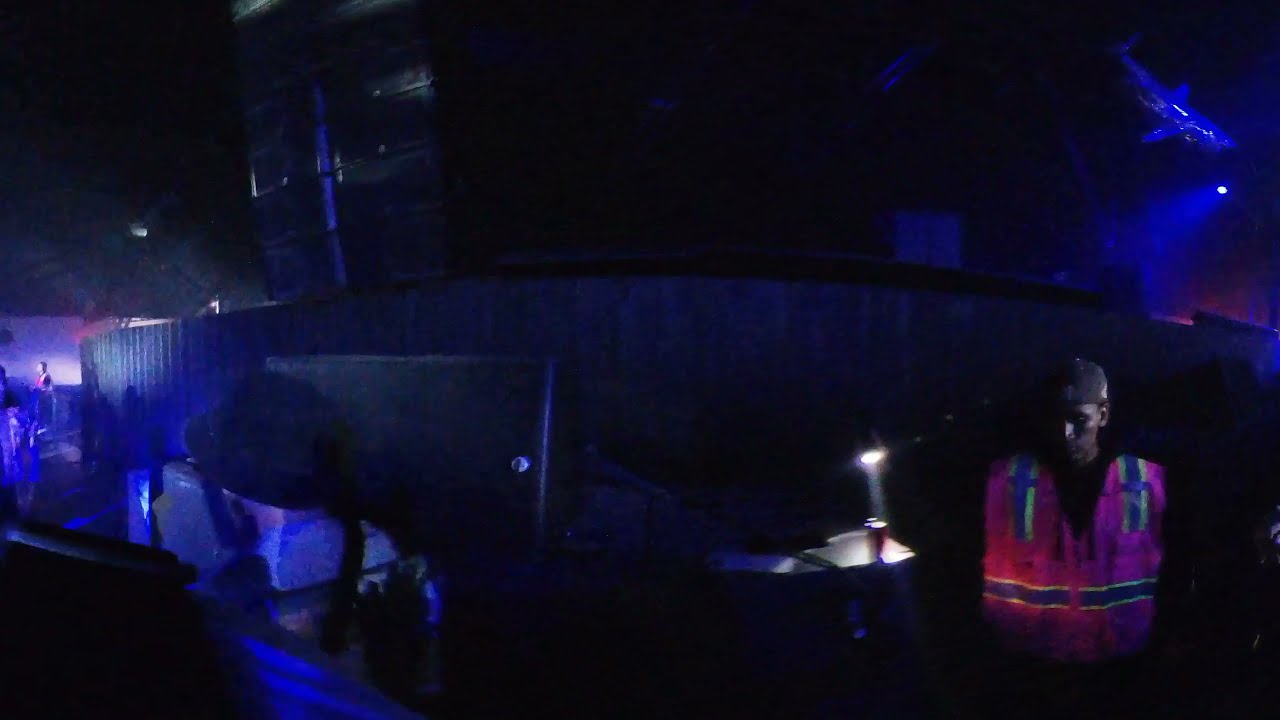The image depicts a dimly lit indoor scene, resembling a nightclub or the backstage area of a concert. The top portion of the image is enveloped in darkness, with subtle blue highlights creating a mysterious ambiance. As the view descends towards the bottom, faint lighting reveals more details. On the left side, the scene is slightly illuminated, exposing blurry objects including a white planter, mannequins, and some lighter purple areas. 

In contrast, the right side of the image is dominated by a spotlight that illuminates a small table and a man standing nearby. He is wearing a bright orange or red high-visibility vest, adorned with blue and lime green light-up stripes, typical of a construction worker. He also wears a dark-colored hat and appears to be looking downward, focused on an object or screen below him. Besides him, there appears to be a flashlight that is casting light. Above this man, a floating shark decoration adds an unusual element to the scene.

Overall, this panoramic view down a corridor, reveals a quiet and enigmatic environment, suggesting settings of either a nightclub or a concert’s backstage area.